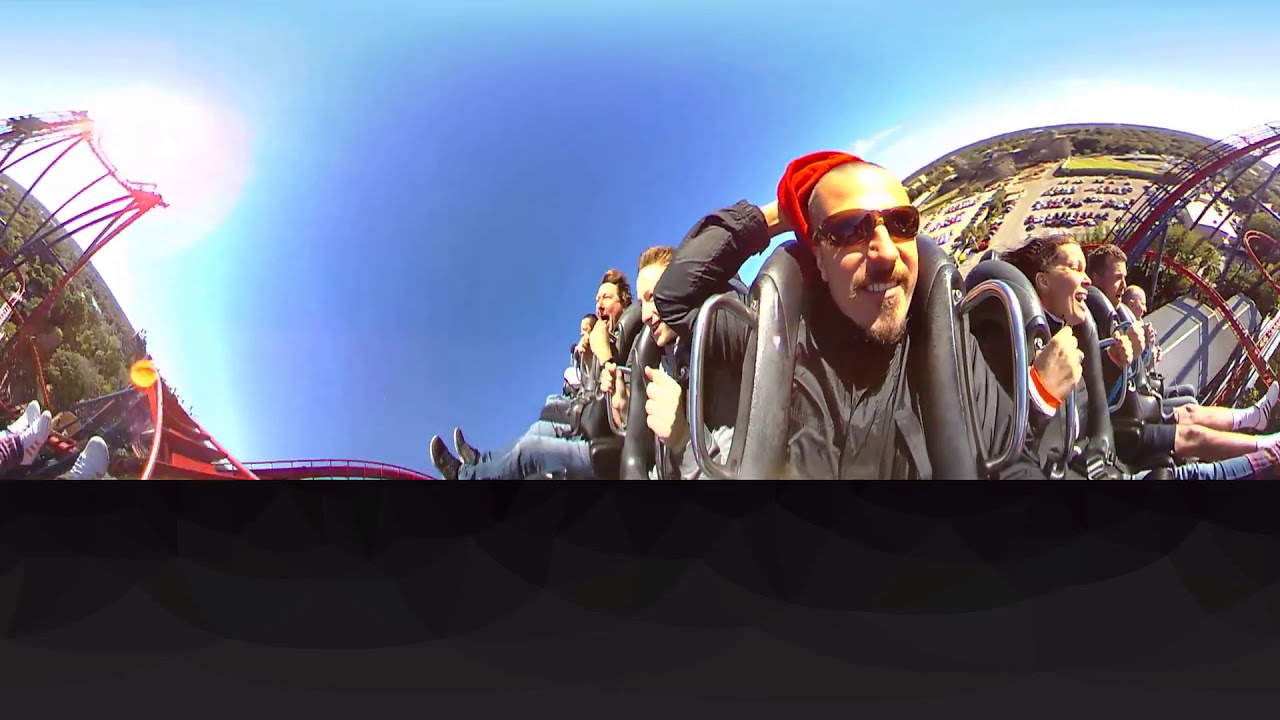A bright, sunlit day at the amusement park is captured in this dynamic fisheye lens photo taken from a roller coaster. The image, slightly distorted due to the fisheye effect, features a man as the central figure, seated with a rubber black harness across his shoulders and silver handlebars in front of him. He is holding onto a red beanie with one hand to prevent it from flying off, his short hair visible beneath it. Wearing sunglasses, the man smiles widely, his goatee and mustache casting a slight shadow in the intense sunlight.

Surrounding him are six other riders, all strapped into their seats, with expressions ranging from laughter to screams as they experience the thrill of the ride. Their hair is blown back by the wind, and their legs stretch out in front of them, gripping the bars for dear life. On both the left and right sides of the image, the roller coaster's red track curves and loops, adding to the sense of exhilaration and chaos.

The background displays a bright blue sky without a cloud in sight, suggesting a clear and vibrant day. Below the coaster, a parking lot filled with cars and a lush forest area can be seen, adding to the overall scene's depth and context. Despite the high-angle view and the fisheye distortion, the photo vividly captures the excitement and energy of a roller coaster ride, with the man and his fellow riders epitomizing the joy and thrill of the moment.